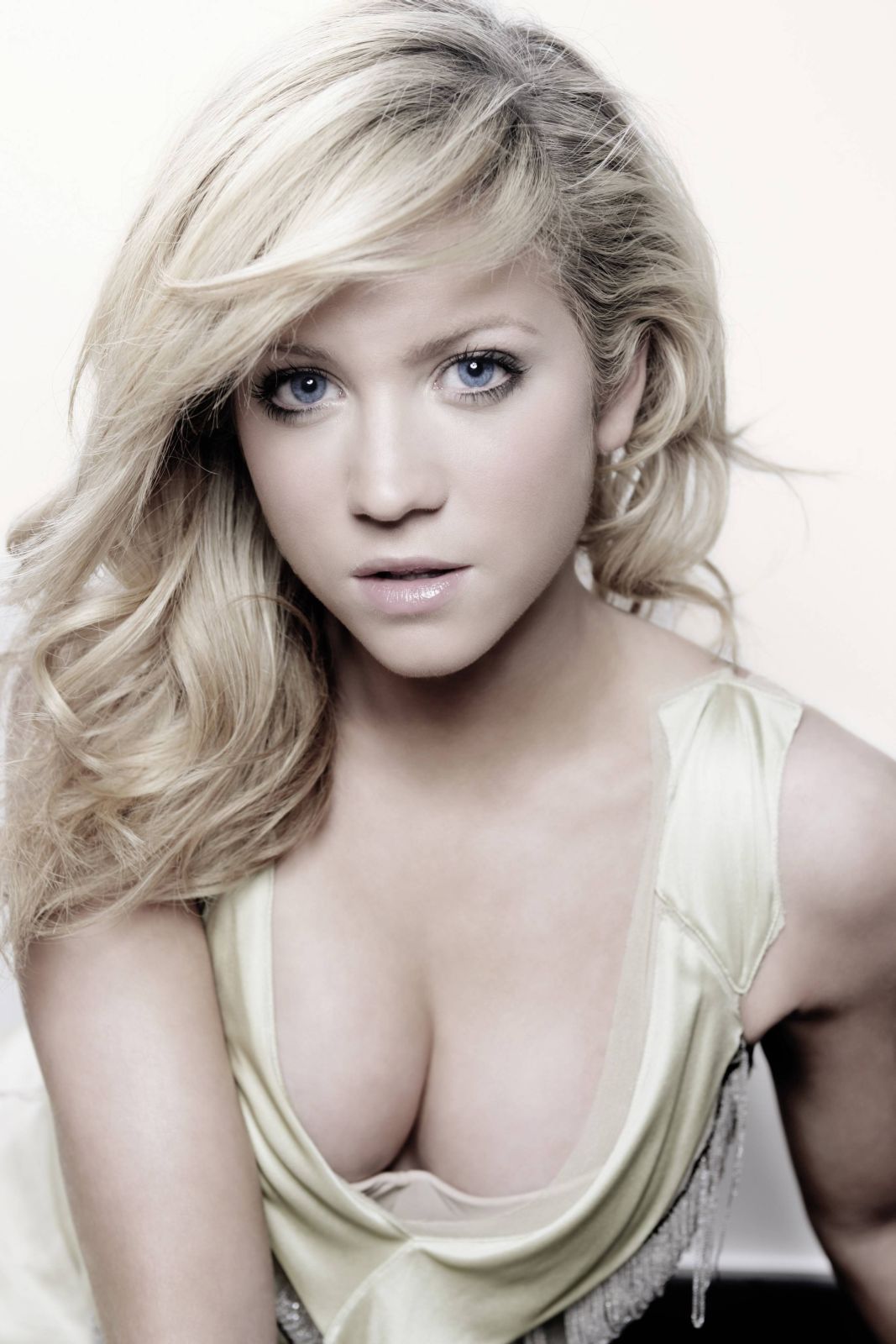The image shows a close-up view of a young woman with wavy blonde hair that is pulled to one side, cascading down to about her shoulders. She has blue eyes and white skin, and she's looking directly ahead with her mouth slightly open, though not smiling. She is wearing a very low-cut, yellowish-green dress with very thin straps, exposing the top of her chest and the upper parts of her arms. The background of the picture is a light, ivory color, providing a soft contrast to her attire. The photograph is vertically oriented and rectangular in shape, capturing her from just below the chest upwards. There appear to be small fringes on the lower right-hand corner of her dress.